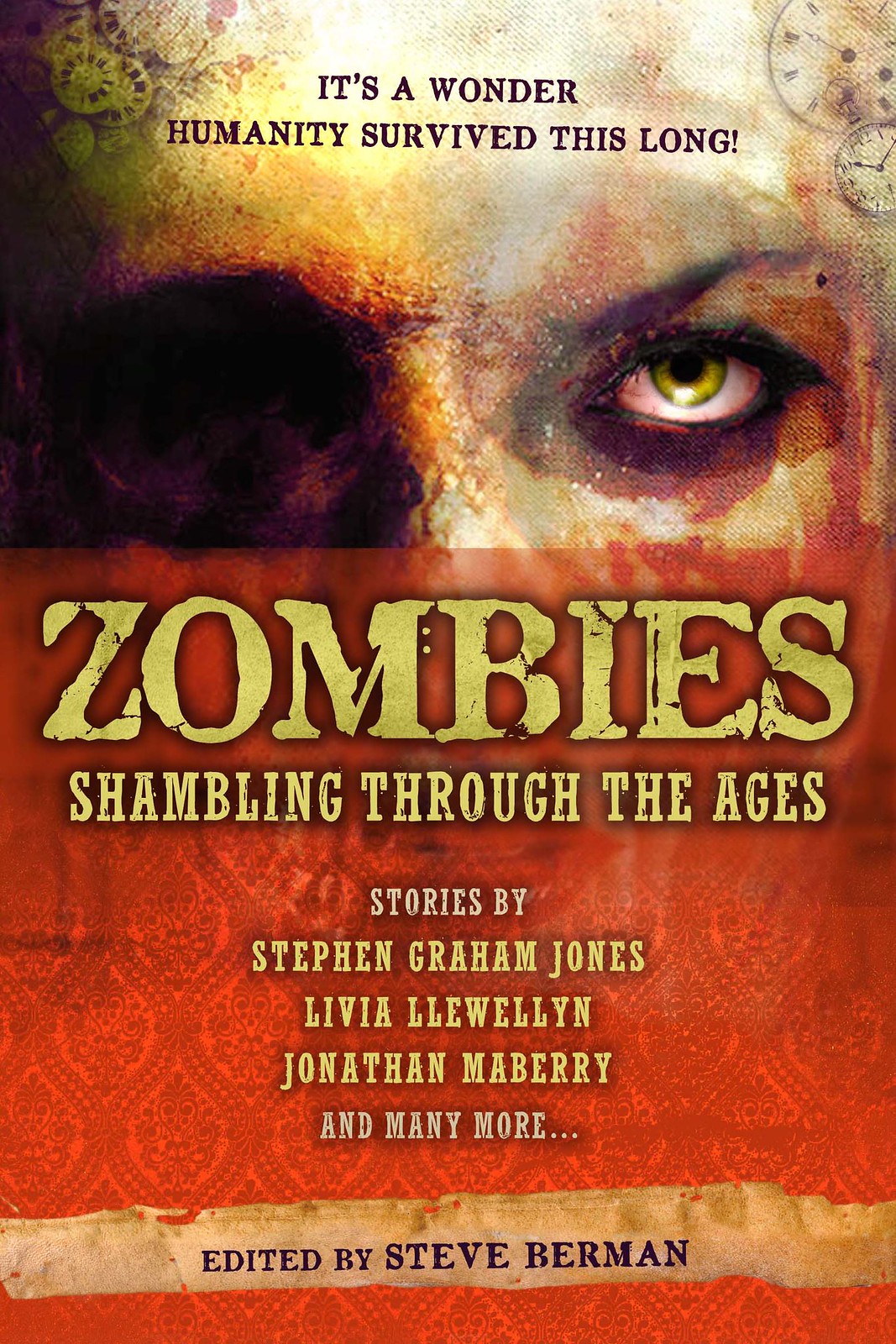The image depicts the cover of a captivating book titled **"Zombies: Shambling Through the Ages."** The title is prominently displayed in bold yellow letters across the center of the cover. The background exudes a harrowing, eerie atmosphere with hues of orange and reddish tones. At the very top, an ominous caption reads, *"It's a wonder humanity survived this long."* 

Beneath this headline, the focal point features a haunting visage of a zombie. The eyes capture significant attention; the left eye socket appears purple, resembling a skull, while the right eye, though almost normal in shape, is olive green with unsettling red and yellow splotches. 

Below the image of the zombie, the banner continues with crucial information about the book's contributors. The names **Stephen Graham Jones, Livia Llewellyn,** and **Jonathan Maberry** are listed as authors, with the phrase *"and many more..."* hinting at additional contributors. At the very bottom, a banner declares, *"Edited by Steve Berman."* This detailed cover design effectively sets the tone for the macabre tales contained within the book.